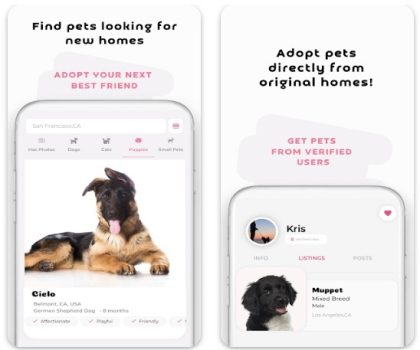The image depicts two sections of a website interface designed to facilitate pet adoption. 

On the left side, there is a rectangular area titled "Find Pets Looking for New Homes" in black text, with a subheading "Adopt Your Next Best Friend" in red text beneath. Below this, there is an outline of the top and middle part of a cell phone, followed by an open search bar. Underneath the search bar, there is an image of a German Shepherd puppy with floppy ears adorably hanging to the side.

On the right side, there is another rectangular section. The top of this box reads "Adopt Pets Directly from Original Homes" in black text, followed by "Get Pets from Verified Users" below. Underneath this, there is an image showing the top half of a cell phone. On the top right corner of the phone screen, a favorites bar is visible with a heart highlighted in red, indicating a favorited item. On the left side of the phone screen, there is a circular icon with an image of a person holding a dog on a leash. Beside this icon, the name "Chris" is displayed. Further down, there is a picture of a black dog with floppy ears, slightly panting with its mouth open, showing its tongue, and having a white patch on its chest. To the right of the dog's image, the name "Muppet" is displayed along with "Mixed Breed Male."